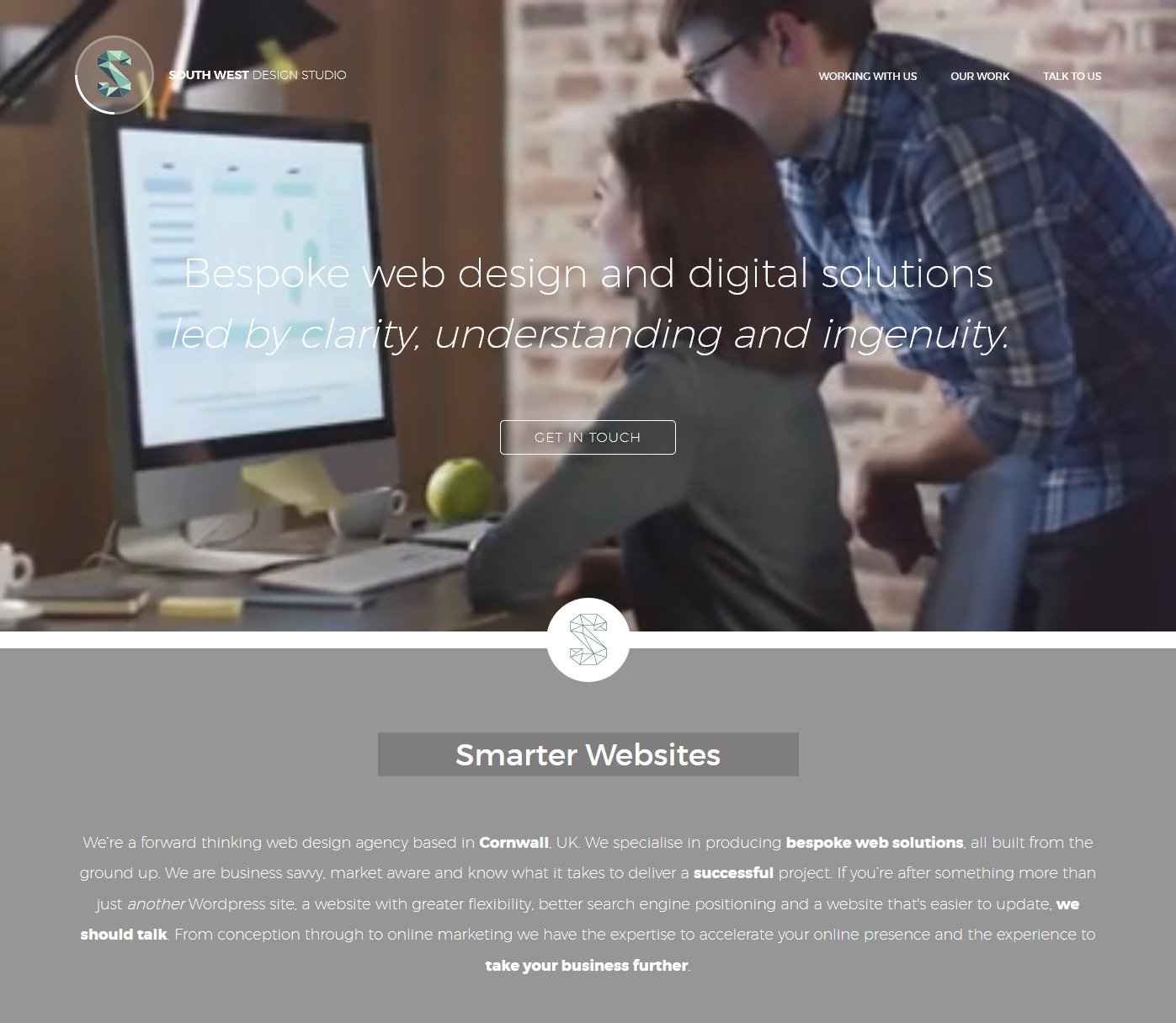The advertisement for Southwest Design Studio features a professional setting with a focus on collaboration and quality web solutions. In the image, a woman dressed in a grayish-green shirt is deeply engaged at her computer, supported by her elbows. Her workspace includes a literal apple, a small coffee cup, and some scattered notes, suggesting a productive environment. Behind her, a gentleman in glasses, dressed in a plaid shirt, leans on her desk chair, peering over her shoulder at the computer screen, indicating teamwork and attention to detail.

The Southwest Design Studio logo, prominently placed, is designed to resemble origami paper, adding a creative touch. The tagline at the bottom reads "Smarter Websites." The accompanying text describes the studio as a forward-thinking design agency based in Cornwall, UK, specializing in bespoke web solutions developed from the ground up. The agency prides itself on being business savvy and market-aware, capable of delivering successful projects. Prospects are encouraged to engage with Southwest Design Studio if they are looking for more than just another WordPress site, opting instead for a website with greater flexibility, better search engine positioning, and ease of updates.

Highlighted in bold are the phrases: "We are business savvy, market aware, and know what it takes to offer a successful project," and "If you're after something more than just another WordPress site and a website with greater flexibility, better search engine positioning, and a website that is easier to update, we should talk."

The ad goes on to emphasize their comprehensive capabilities from conception through to online marketing, asserting their expertise in accelerating online presence and the experience to propel a business further. These key points are also presented in bold to capture the reader's attention effectively.